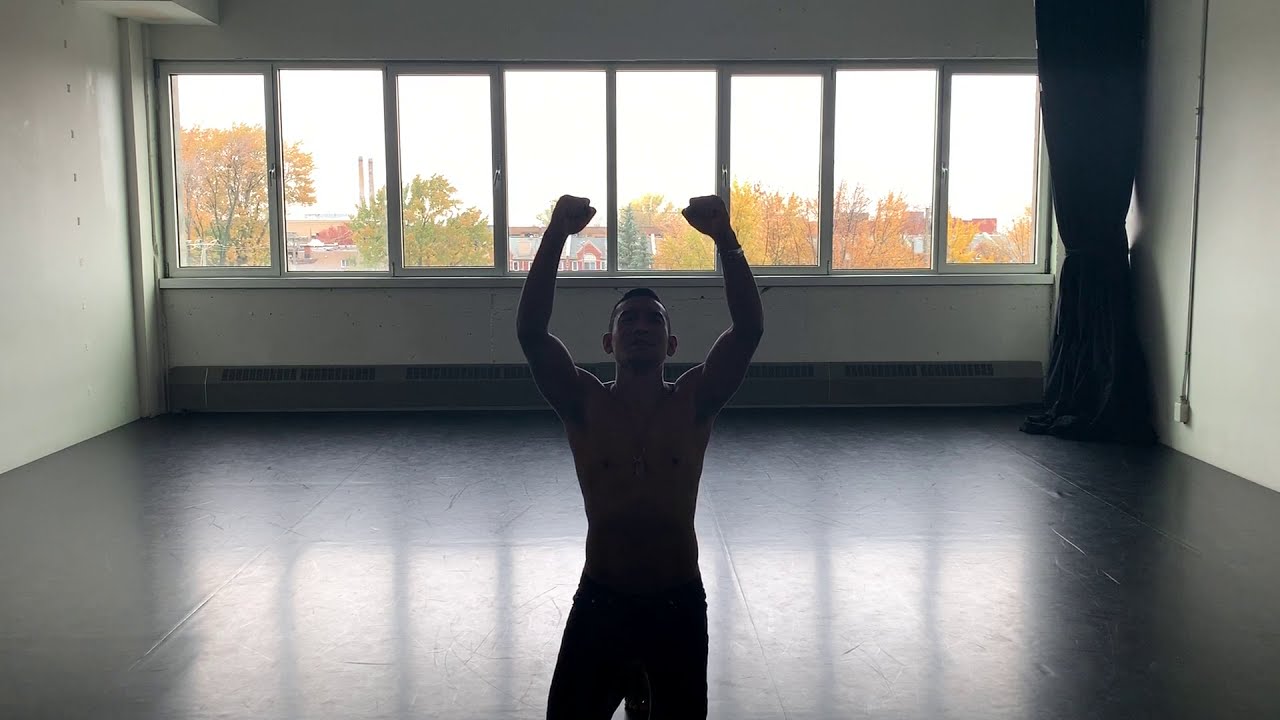The image depicts a shirtless man on his knees in a sparsely furnished studio, hands raised triumphantly. The room is dominated by eight large windows on the back wall, through which natural light floods in, creating a dramatic silhouette of the man. This makes it challenging to discern his features, but his muscular build is evident. The studio's floor is dark, likely brown or black, and there's minimal decoration, enhancing the room's starkness. On the right side of the wall, a large curtain hangs, partially drawn to allow the sunlight to illuminate the space. Outside, trees, buildings, and an expanse of sky are visible, adding a serene backdrop to the otherwise spartan environment. The studio's white walls and the presence of what appears to be a vent at the bottom suggest it is a functional space, possibly used for dance or yoga.